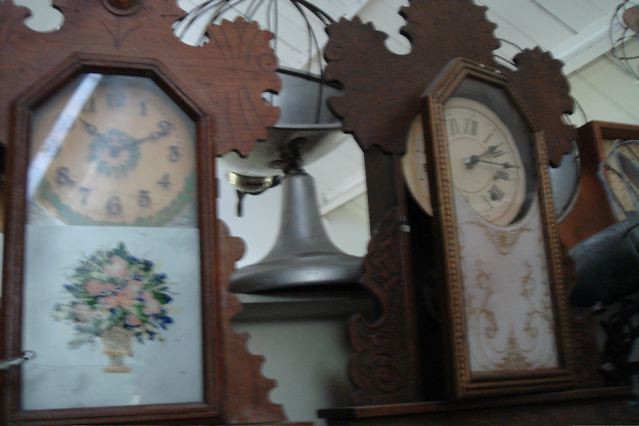This image showcases a close-up view of two ornately designed, old-looking mantel clocks positioned on a shelf. Both clocks have vertical rectangular wooden frames with an intricate trident leaf pattern adorning their top edges. The left clock is slightly lighter in brown hue with a distinctive design—its corners fan out and curve back inwards, resembling the shape of birds with open mouths and visible eyes carved into the sides. The round clock face, bordered in green and set behind a glass panel, features yellow in the center and black hands. Below this, a white stained glass section displays a colorful painting of a bouquet in a vase with pink, blue, and green accents. The darker brown clock to the right shares a similar decorative bird pattern but with a slight color variation. Its clock face shows Roman numerals and also has a white glass section on the lower half adorned with abstract gold filigree designs. 

In the background, a minimalist decorative globe crafted from black wire and devoid of any map, rests precariously on a silver stand, partially hanging off the edge of the shelf. The environment hints at a farmhouse setting, with visible white painted shiplap rafters and beams on the ceiling, contributing to the rustic ambiance of the scene. Additionally, the top left corner of another brown clock just peeks into the far right of the image.